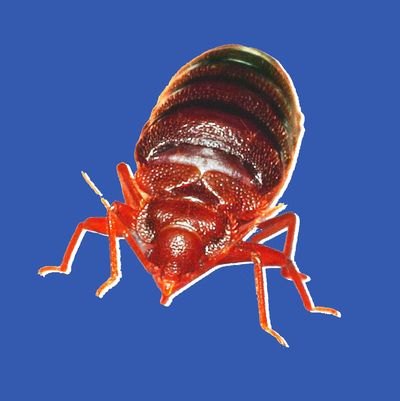The image features a reddish-brown beetle set against a royal blue background. It is a somewhat close-up, top-down view, focusing on the beetle albeit with slightly blurry details. The beetle has a darker brown abdomen adorned with black stripes, and a small head equipped with large eyes and antennae. Each side of the beetle's head displays three legs, with a small mouthpart visible at the front. Light reflects off its face and body, creating a subtle white sheen. The head of the beetle is pointed towards the camera, emphasizing its bulbous, shell-like body. There are tiny circle bumps on its surface, and hints of a white outline around the legs, suggesting that this cropped photograph originally came from a larger image.